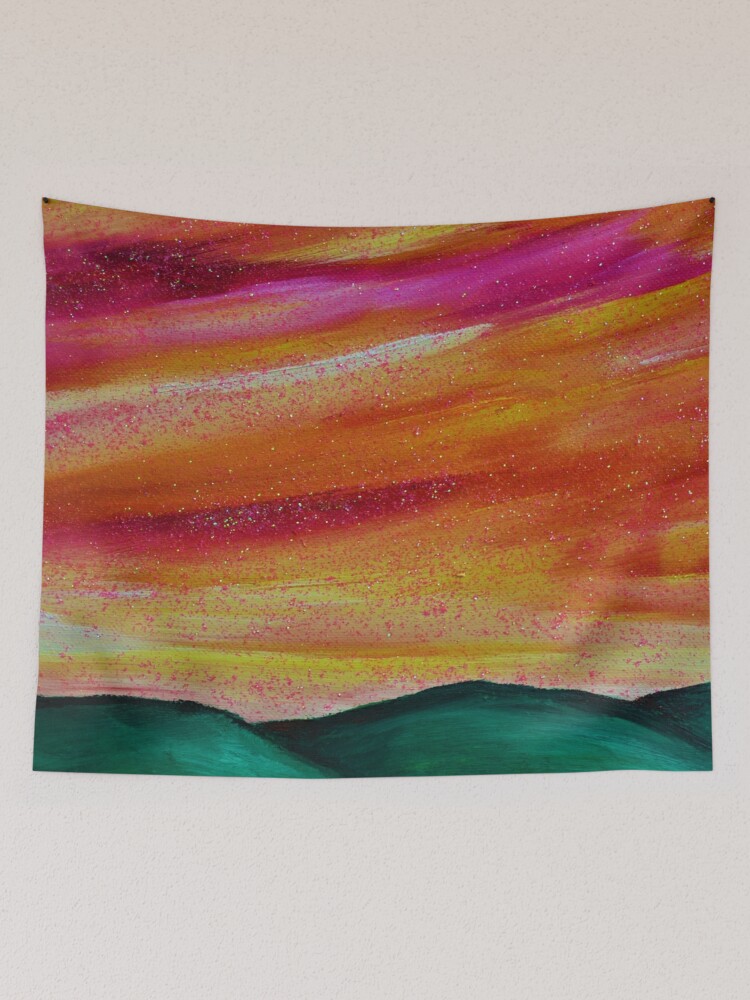Centered on an off-white, light-colored background, there's a square canvas art piece seemingly tacked at the upper corners with two small black dots. The painting, captured in a rough, vibrant style, appears to depict a natural landscape, likely at sunrise or sunset. The lower third showcases dark teal or turquoise-green hills, rendered in broad, rough strokes. Above the hills, the sky transitions through layers of rich colors: deep pinks, almost reds, bold yellows, and fiery oranges, suggesting the sun's last or first light. Specks and swipes of white and pink dots are scattered throughout the composition, adding texture and depth to the colorful brushstrokes. The overall image evokes a vivid, almost abstract interpretation of a sky brilliantly lit with warm hues, blending harmoniously with the serene, dark hills below.